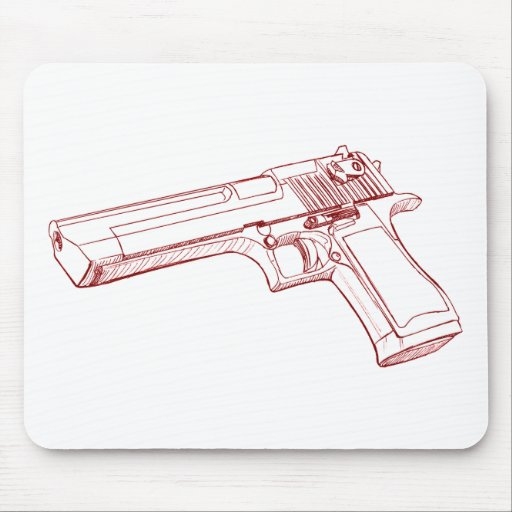The image features a sketch of a white handgun with intricate red outlines and details, set against a predominantly white, wood-textured background. Central to the composition is a square with rounded edges, lighter in color and featuring subtle striations suggesting it may also be wood. Within this square is the detailed drawing of the handgun, depicted with various notable features: a square barrel end, a small hole for the bullet, a trigger in the unpulled position, a safety latch on the top right, and a grip with a large rectangular detail in the middle. The back butt of the gun has visible lines, and there is a hammer towards the rear. The lower part of the gun shows slight shading, adding a three-dimensional effect to the sketch. The overall depiction suggests it may resemble a Glock, with careful attention to elements like the handle, trigger, and barrel.